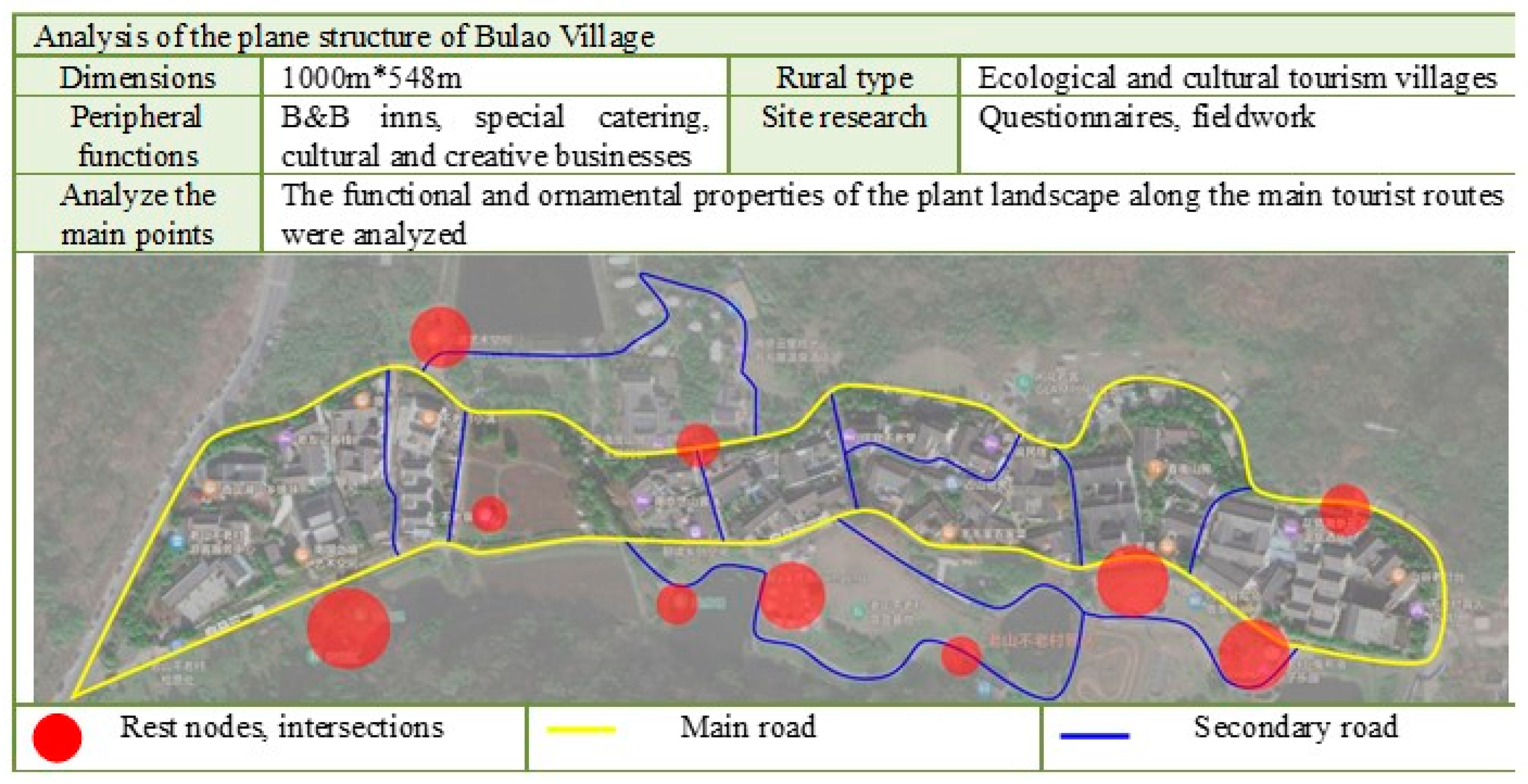The rectangular image measures approximately five inches wide by three inches high, featuring a detailed layout and descriptive analysis of Bulao Village. A green border frames the top and left, while a black border runs along the bottom, leaving the right side open. The caption within the green border at the top reads, "Analysis of the Plain Structure of Bulao Village," with a detailed breakdown below. 

- **Dimensions:** The village spans 1,000 meters by 548 meters.
- **Rural Type:** Bulao is an ecological and cultural tourism village.
- **Peripheral Functions:** Key activities include B&B, special catering, and cultural and creative businesses.
- **Site Research:** Conducted through questionnaires and fieldwork.
- **Analysis Main Points:** Focus on the functional and ornamental properties of the plant landscape along the main tourist routes.

The main portion of the image consists of a map overlaid with yellow and blue lines and red circles. A key at the bottom clarifies that red circles represent rest nodes and intersections, yellow lines denote main roads, and blue lines indicate secondary roads.